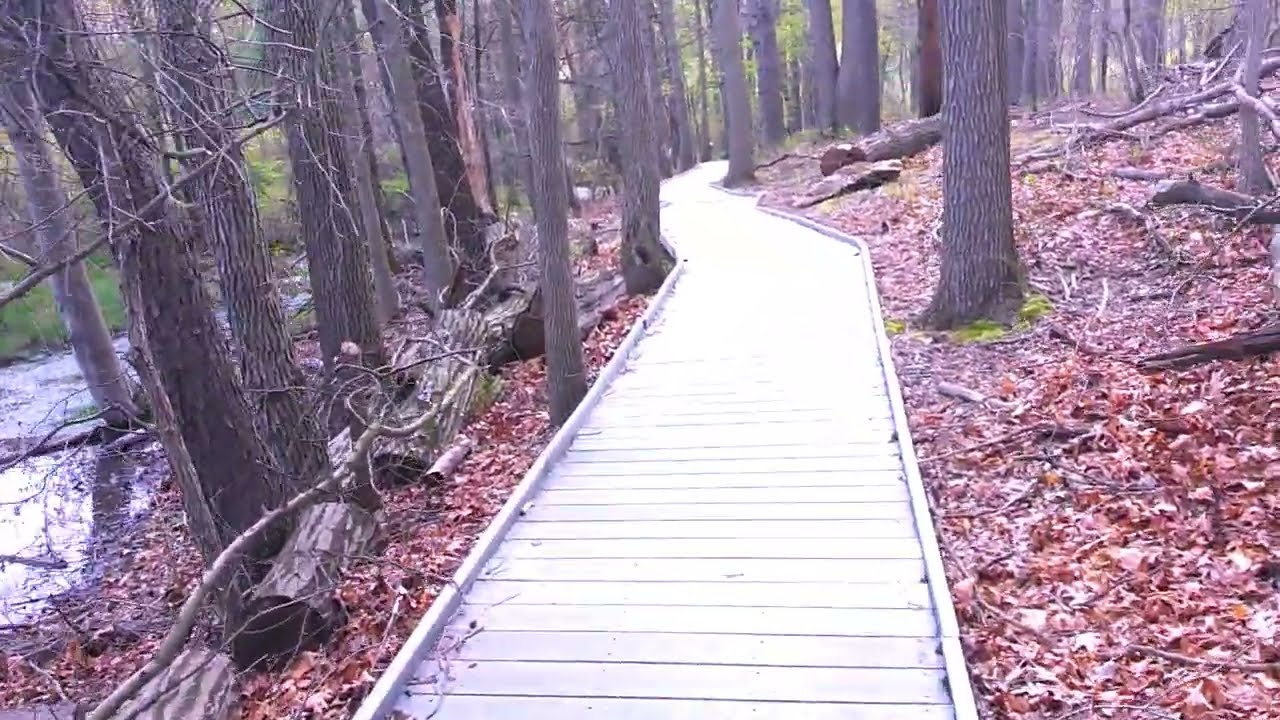The image depicts a slightly faded full-color photograph taken outdoors during the daytime in a wooded area, either in late autumn or early winter. A slatted wooden walkway, appearing almost white and constructed from planks of wood, serves as the central focus of the scene. The pathway meanders through the forest, initially going straight before bending left and then curving back to the right as it follows the natural contours of a hillside. 

Surrounding the path, the ground is blanketed with brown, fallen leaves and dead branches, indicative of the season. To the left side of the path, there is some standing water, possibly a small creek or shallow river, hinting at recent rainfall. The creek is accompanied by downed pieces of trees and logs that appear to have been deliberately cut and placed.

The majority of the trees' trunks visible in the image are bare, lacking leaves, with some green ground cover and leaves visible in the distant background. This contrast between the bare foreground trees and the greener vegetation at the far end of the path adds depth to the scene. Overall, the wooden path invites the viewer to journey into the tranquil, leaf-strewn forest.